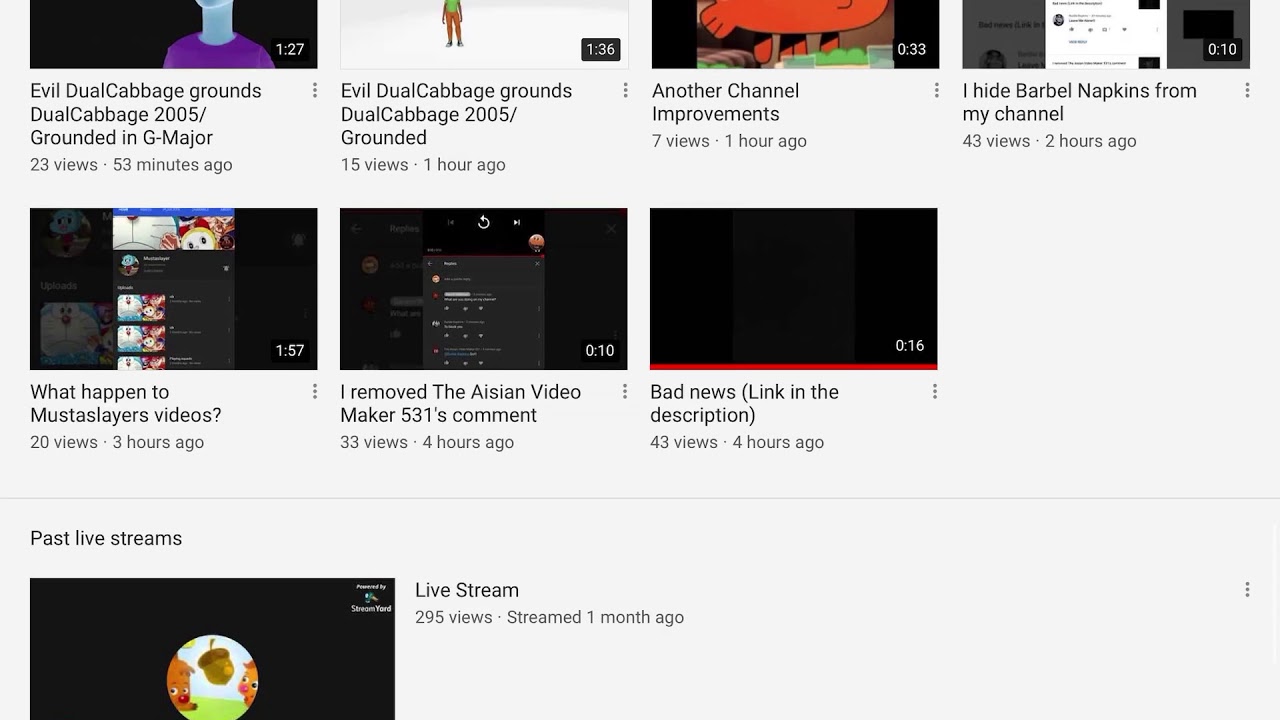The image is a screenshot of the YouTube homepage. At the top left, the first video title visible is "Evil Dual Cabbage Grounds Dual Cabbage 2005 / Grounded in Gene Major." The second video displays a similar title. The third video is titled "Another Channel Improvements," and the fourth reads "I Hide Barbell Napkins from My Channel."

In the second row, the first video is titled "What Happened to Musta Slayers Videos?" followed by "I Remove the Thing is Supposed to Say Asian but They Spelled It Very Wrong - Video Marker 531's Comment." The last video in this row is titled "Bad News" with "Link in the description" noted in parentheses.

At the very bottom, there is a section labeled "Past Live Streams," with an indication of a live stream.